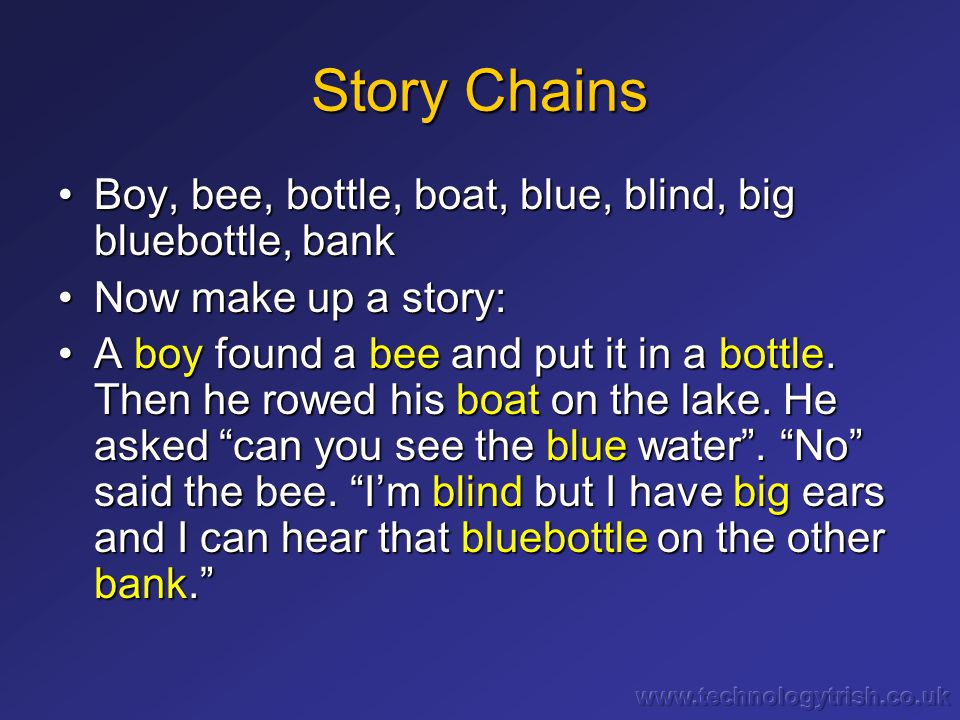The image depicts a PowerPoint slide with a gradient background transitioning from dark blue at the top to a lighter blue at the bottom, accented by distinguishable gradient lines. At the top, the header "Story Chains" is written in a simple, gold Arial font. Below, the slide presents three main bullet points. The first bullet point lists words: "boy," "bee," "bottle," "boat," "blue," "blind," "big," "blue bottle," and "bank." The second bullet point instructs to "Now make up a story." The third bullet point features a narrative:

"A boy found a bee and put it in a bottle, then he rowed his boat on the lake. He asked, 'Can you see the blue water?' 'No,' said the bee, 'I'm blind, but I have big ears, and I can hear that blue bottle on the other bank.'"

In the story, key words such as "boy," "bee," "bottle," "boat," "blue," "blind," and "big" are written in yellow, aligning with the initially listed words. At the bottom right corner, there's a faint, embossed watermark: www.technologytrish.co.uk. The overall slide layout ensures that text is well-positioned with no overlapping.